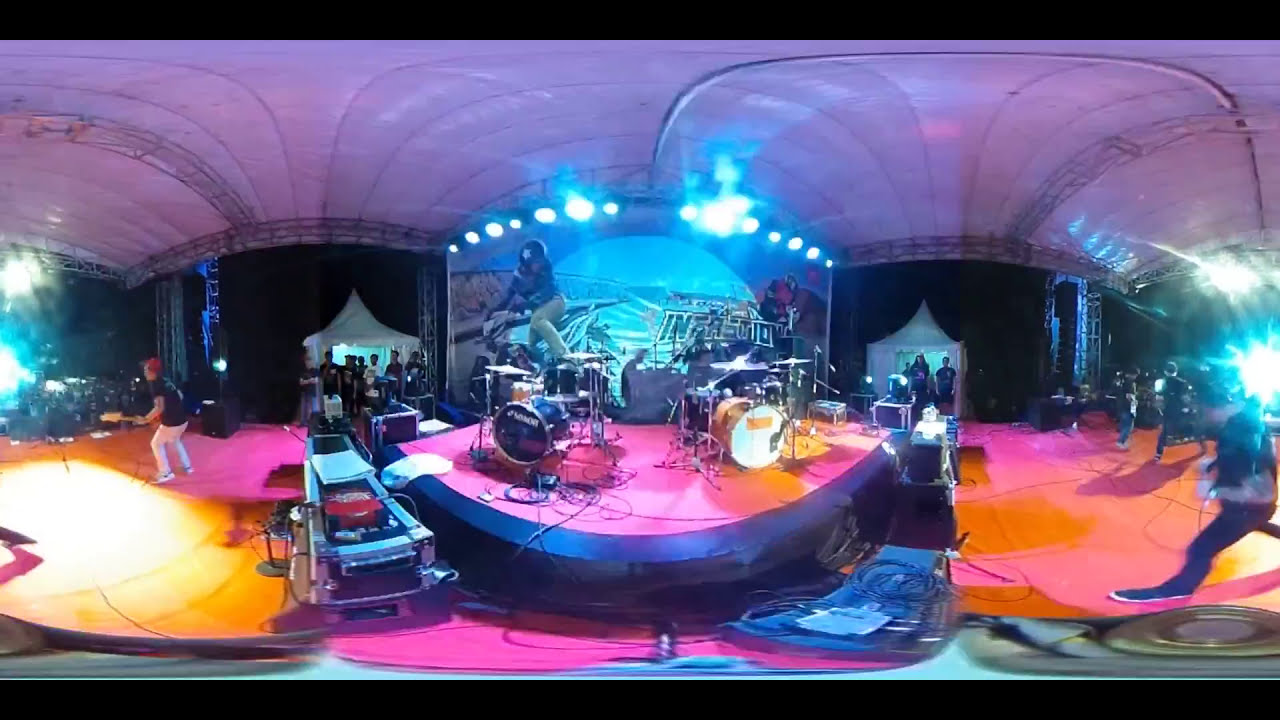This image features an indoor concert venue bathed in vibrant colors of purples, pinks, yellows, and blues, giving it an artistic, almost hand-painted vibe. The focal point is a raised stage covered by an off-white canopy, adorned with numerous colorful lights. Dominating the stage are two drum sets positioned at the front. On the left side of the stage, a guitarist in white pants and a black shirt, with a red baseball cap, faces away from the camera. Further to the left, additional equipment is visible. On the right side, a group of people stands idly, with one person seemingly running towards the stage, somewhat obscured by bright light. Additionally, towards the right and further back, beneath white and black curtains, more individuals are gathered, adding depth to the scene. Behind the stage, a wall features circular lights, and a backdrop projection seemingly depicts people riding motorcycles. The text "I-N-T-R-F-A-S-O-I-D-U-S-T-I-O" is faintly legible, suggesting either a decorative or thematic element. The foreground includes a table with an indistinguishable red object atop it, positioned before a dividing wall that separates the stage from a potential dance area. The eclectic and bustling scene hints at a rehearsal or an ongoing performance, encapsulating the dynamic atmosphere of a lively entertainment venue.